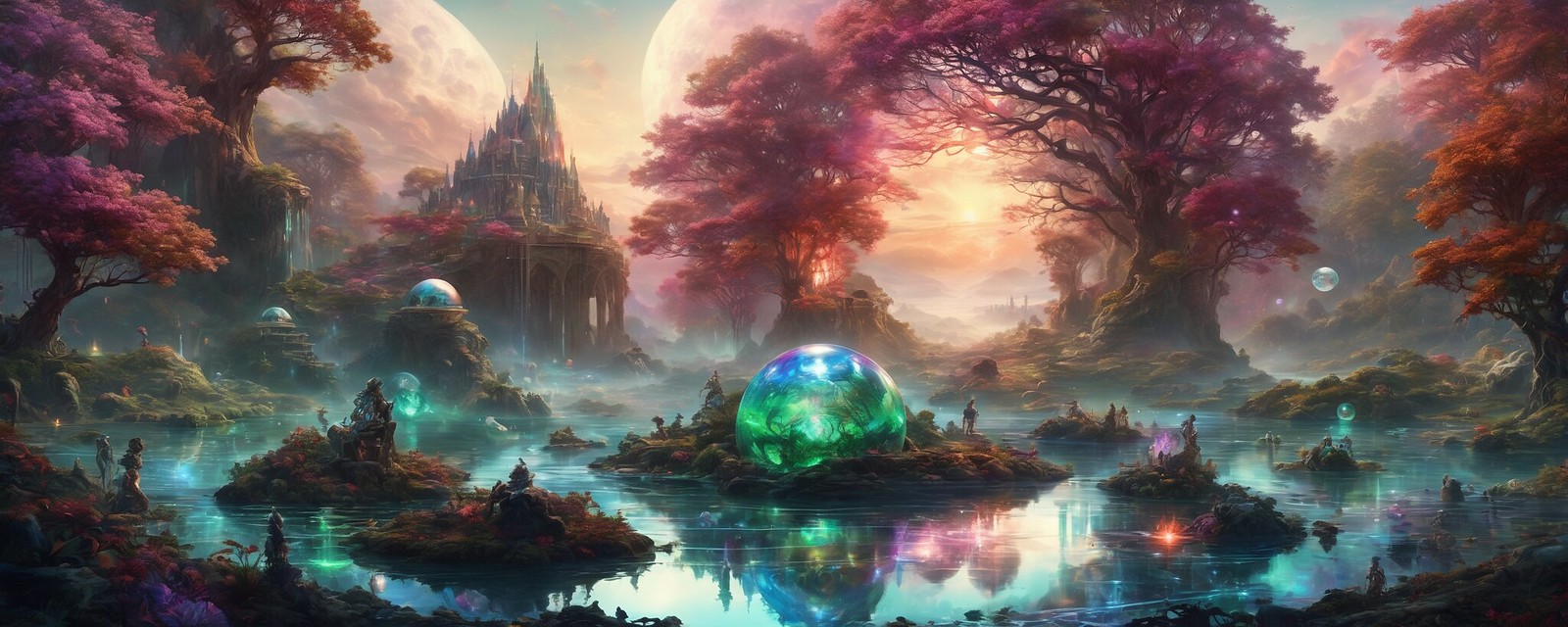This fantastical painting is a horizontal and thin composition depicting an otherworldly scene. Central to the artwork is a glowing greenish-blue orb situated on a rocky outcrop in the middle of a highly reflective lake, whose waters ripple gently. Surrounding this central feature are small mounds and outcrops of land. The scene is populated with humanoid figures scattered around the shore and on the islands, gazing toward the mysterious glowing orb.

The background is dominated by a grand castle with numerous towers, perched on a floating rock or cliff side. This is complemented by columns resembling icicles, adding to the fantasy element. The sky above features two moons and clouds that are almost moon-like in their circular shape, imparting an ethereal atmosphere to the painting.

The landscape includes trees with striking, pinkish-red leaves, some with wide bases that could either be part of their trunks or the earth below. Among these are both pink and orange-leaved trees, creating a vivid and colorful setting. Additionally, floating bubbles and smaller glowing orbs appear throughout, enhancing the fantastical feeling. Overall, this painting captures a magical, dream-like world filled with whimsical details and vibrant, otherworldly beauty.